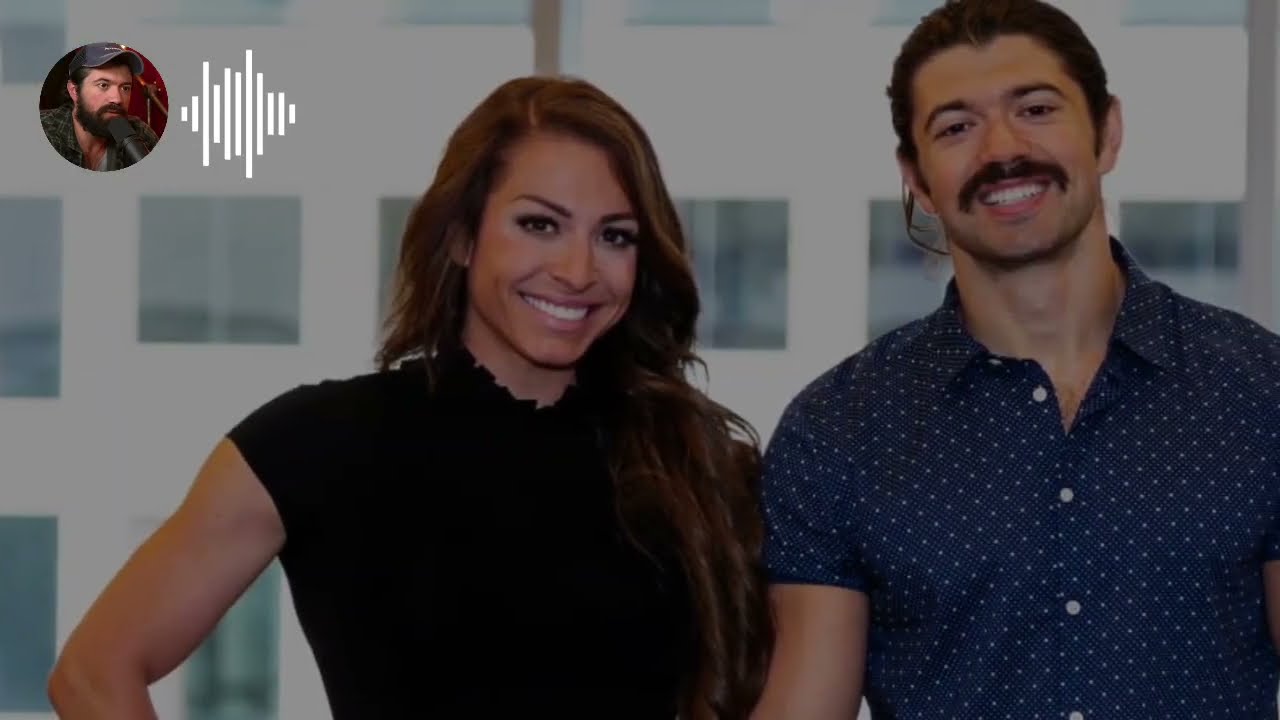The image features a young man and woman, both appearing to be in their thirties, standing close together. The man, situated on the right, is wearing a dark blue short-sleeve button-up shirt adorned with white polka dots, and he has his dark brown hair pulled up into a bun. He sports a mustache and is smiling at the camera. There's an item, possibly a wire or a microphone, hanging from his ear. The woman, on the left, has long, wavy brown hair that cascades down to her chest, and she's wearing a black blouse with a ruffled neckline. She is also smiling brightly, showcasing her white teeth. Her right arm is extended with her hand resting on her hip, indicating a relaxed posture. The background is slightly blurry, revealing a white building which appears to be part of a backdrop, with some light green squares visible on the wall behind them. In the upper left corner of the image, there's an inset circle featuring a man with a beard and a hat, alongside a sound bar icon, suggesting that this is a screen capture from a reaction video.